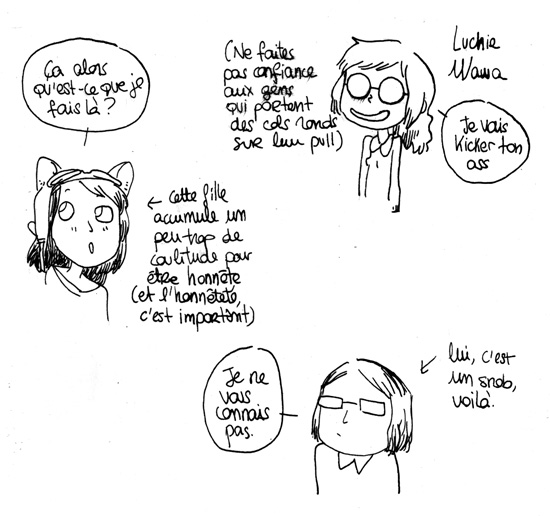The image is a hand-drawn cartoon sketch from a blog titled "Misadventures of Elly, the PhD Student Triathlete." It features three characters, each drawn in black and white against a solid white background. The characters are positioned with one in the center left, and the other two in the top right and bottom right corners. Surrounding the characters are speech bubbles written in handwritten French, making the text somewhat difficult to read. However, translations reveal some of the dialogue, including phrases like "What do they do there?", "No mistrust to the people," "I love the sweater," and "There you go." The characters appear to be discussing various scenarios related to their situations, adding to the comic's narrative. The style and setting of the image suggest it is part of a hand-drawn comic series.